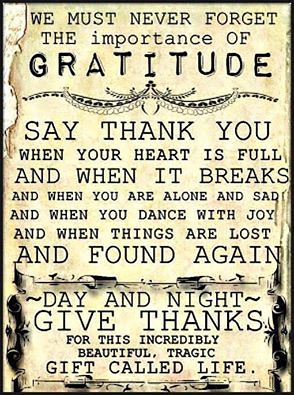The image depicts a vintage-style sign with an aged, ivory or sepia-toned background, designed to resemble old, worn paper. The top left corner is illustrated to appear curled and torn, adding to its antique look. Surrounding the text are stylized edges, mimicking burn marks or black dirt, enhancing its old-fashioned charm. The sign prominently features the word "Gratitude" in bold letters, just below which is a decorative mustache-like pattern or ribbon design that separates the introductory phrase from the body text. The message on the sign reads: "We must never forget the importance of gratitude. Say thank you when your heart is full and when it breaks, and when you are alone and sad, and when you dance with joy, and when things are lost and found again. Day and night, give thanks for this incredibly beautiful, tragic gift called life." This poignant and reflective quote is framed within the visually weathered edges, giving it an evocative and timeless feel.